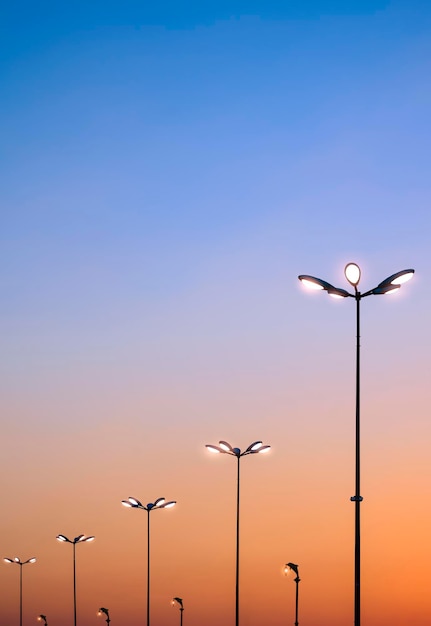This is a color photograph taken outdoors that captures a row of illuminated streetlamps set against a beautiful sky at dusk. The focus is on the streetlamps, resembling those found in a parking lot. The image features a total of nine lampposts arranged in two rows: the front row consists of five tall lampposts with clusters of five glowing lights each, while the back row contains four shorter poles with single lights. The lampposts appear as black silhouettes against the sky. The sky itself is a captivating gradient, transitioning from a baby blue at the top to a warm orange hue near the horizon, indicating the sun is setting. The ground is not visible in the image, ensuring all attention is drawn to the striking contrast between the glowing lamps and the vibrant sky. There is no text or additional elements in the photograph, allowing the viewer to fully appreciate the serene and colorful scene.